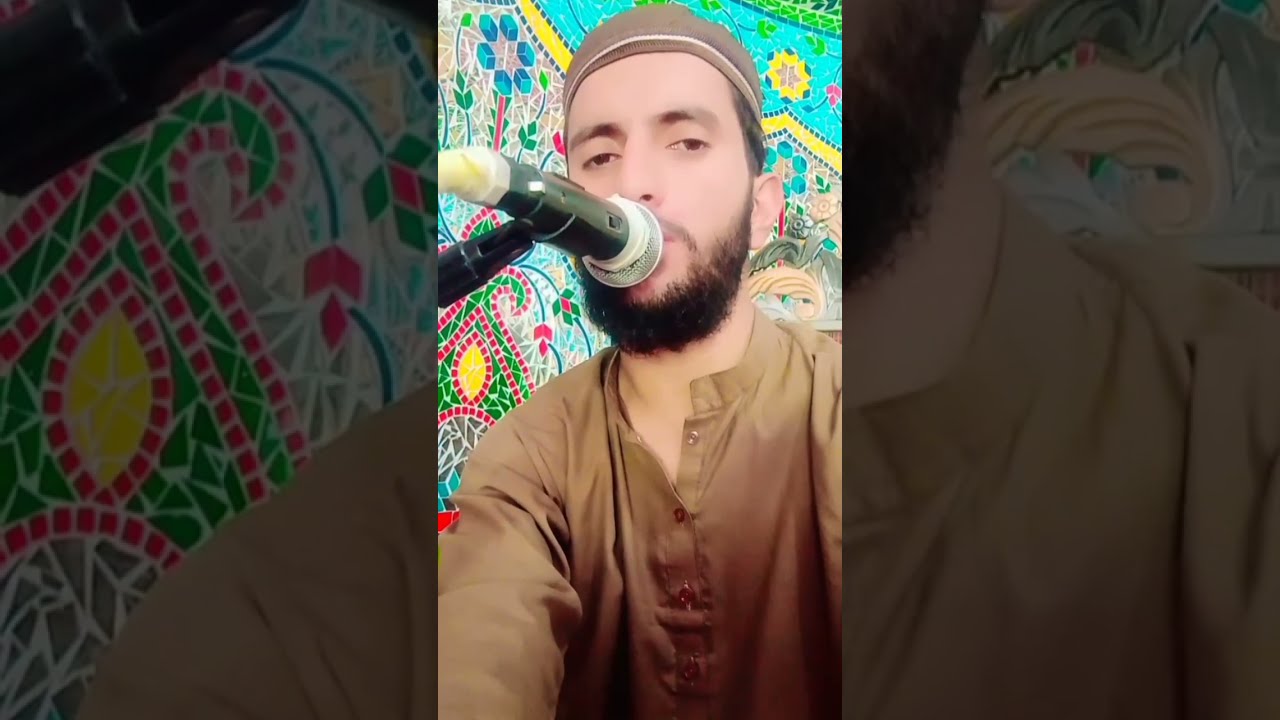This detailed image depicts a man with a beard and mustache, wearing a tan long-sleeved button-up shirt with the top button undone, and donning a knit cap. He is actively speaking or possibly singing into a large microphone that partially obscures his mouth and the right side of his face. His eyes appear to be looking downward, giving his eyelids a partially closed appearance. The background is adorned with a vibrant, artsy, and creative mural that features an array of colorful elements, including flowers and stars, in bright hues such as yellow, green, blue, red, pink, and black. This mural provides a lively, quilt-like backdrop to the scene. The photograph is presented in three panels – the central panel showcases the man at the microphone, while the two outer panels are underexposed blowups of the left and right sides of the central image, creating a thick, grayed-out border on both sides. In the mural, specific details like a blue flower with a red stem, a yellow decorative element, and various turquoise, red, and green tiles stand out, enhancing the vividness of the scene.